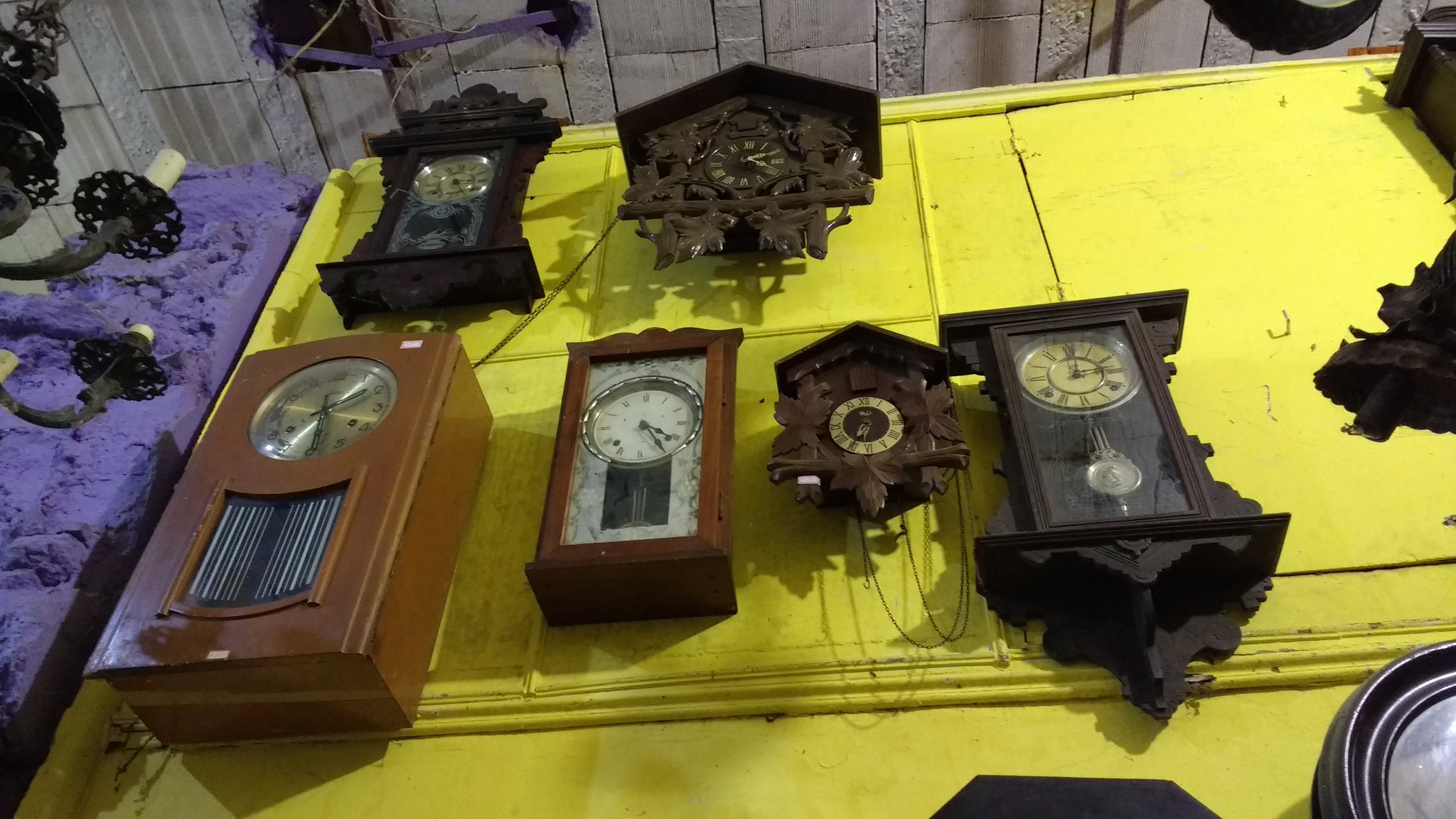This image is a low-angle view showcasing six antique and modern wall clocks hung on a distressed, bright canary yellow wall with faint square patterns. The clocks, varying in shapes and sizes, include a mix of German-style cuckoo clocks and more modern rectangular designs. Dominantly colored in reddish-brown and dark, almost black brown hues, several clocks display their times using Roman numerals. The wall, which appears battered and weathered, is accompanied on the left by a fluffy, purple surface, possibly stones or fabric that extends as high as the yellow wall. Above, the silver or gray ceiling features rectangular drop panels, and in the top left corner of the image, a black chandelier with white candles is partially visible, adding to the antique ambiance. This setting, with its eclectic mix of clocks and aged decor, suggests the image might have been taken in an antique shop or a similar vintage-themed space.